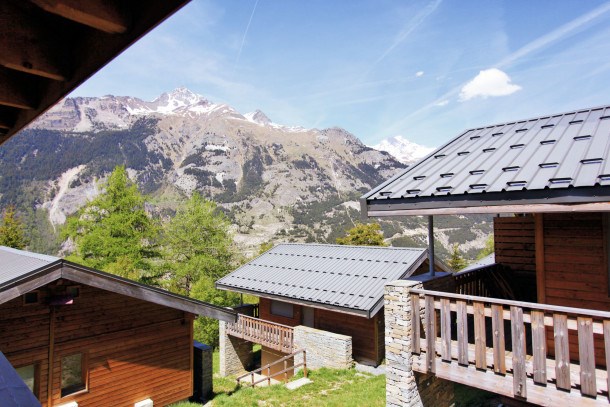The photo captures a scenic hillside landscape featuring three robust, rustic cabins made primarily of wood and stone. These two-story cabins are arranged on a sloping incline, each with distinctive wraparound wooden balconies set against sturdy stone walls. The roofs appear to be covered in gray slate, emphasizing their winter-ready, cold-climate design. The cabins are nestled amidst a green hillside, surrounded by scattered trees. In the background, a majestic, snow-capped mountain looms, with its lower slopes cloaked in dense, dark green trees. The upper part of the image is filled with a light blue sky, tinged with wispy clouds and a touch of mist near the mountain peaks, adding to the serene, picturesque quality of the scene. The vantage point appears to be from the balcony of another similar cabin, highlighting the cohesive architectural style of the area.